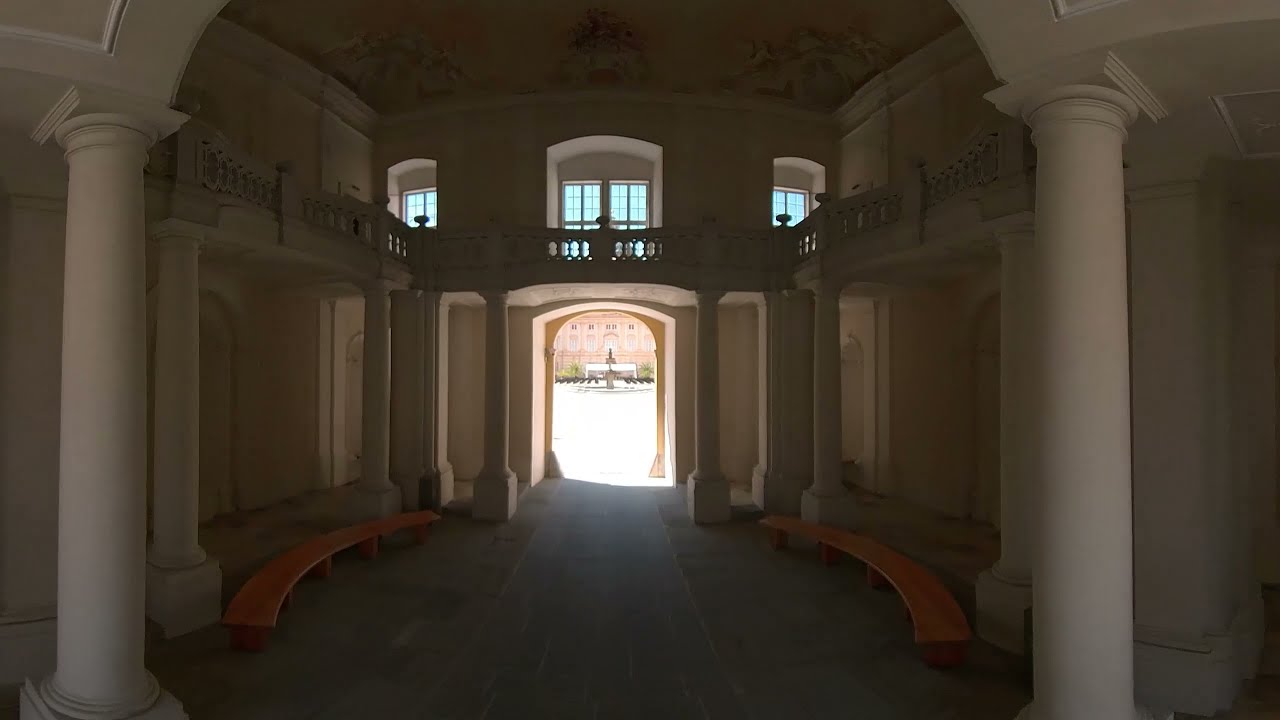The image showcases a highly detailed interior of a grand, possibly ancient building, designed either as a hyper-realistic painting or a photograph. The spacious atrium is accentuated by large, cylindrical columns and rounded wooden benches. This area has a second floor with a stone railing marked by round caps and small windows, allowing in natural light that emphasizes the overall muted palette of black, white, gray, blue, tan, orange, and brown. The interior appears well-crafted with architectural elements that suggest luxury, such as white columns and detailed stonework. Despite this, there's a sense of solemnity as no people are present, enhancing the sense of quiet grandeur. At the center, an open doorway frames a sunlit plaza, hinting at a possibly outdoor fountain and a large building in the background, exemplifying richness and meticulous design. The scene is bathed in subtle daytime light, creating a serene yet somber atmosphere within what could be a sacred temple, a mausoleum, an old house, or even a posh office building.